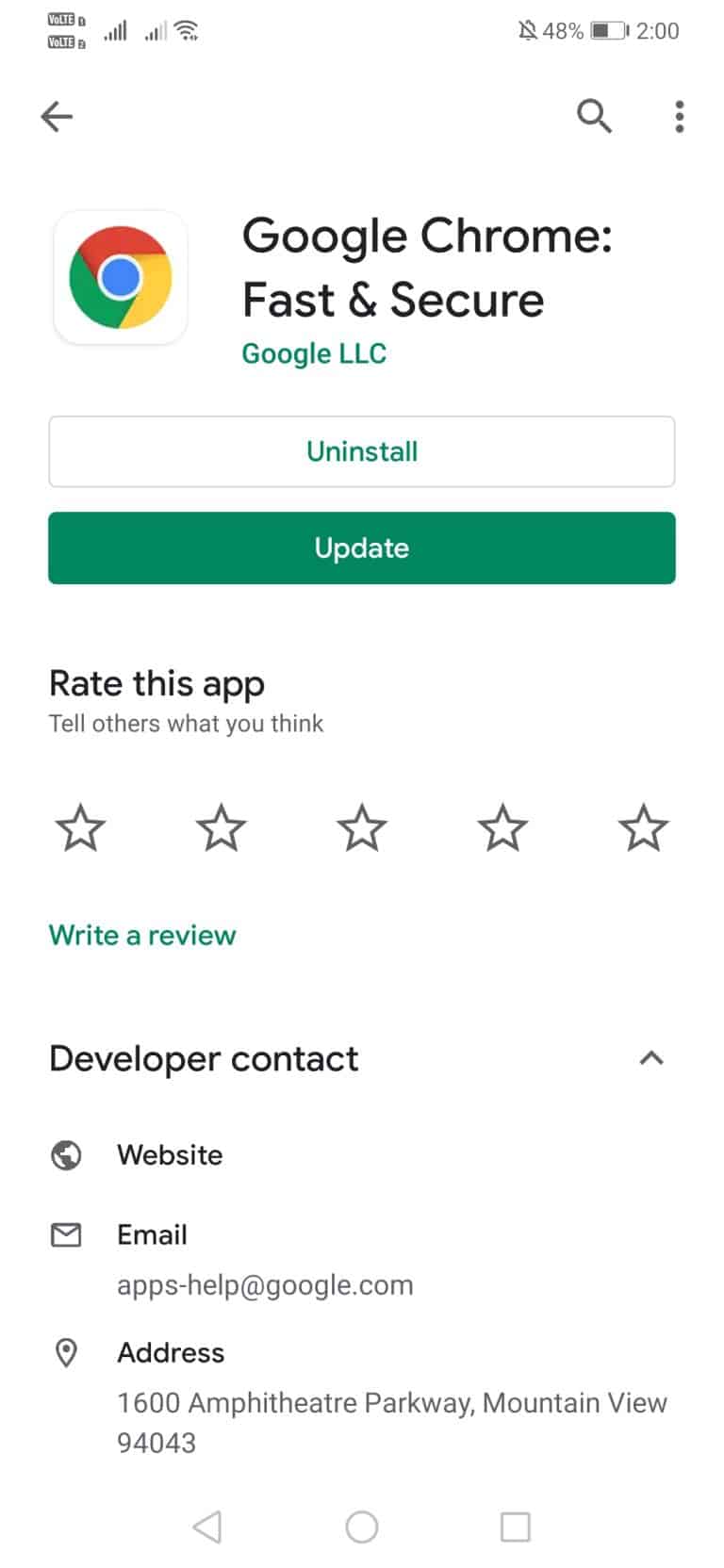Screenshot of a mobile phone depicting the Google Play Store interface for the Google Chrome application. The top left corner of the screen features an all-white background. Two rectangular indicators display "V-O-L-T-E" in black and white lettering, one with a white number "1" in a small square beside it, and the other with a black number "2" beside it. The signal strength indicators show five full bars, another with three out of five bars, and the Wi-Fi strength is full. The sound is muted, indicated by a sound icon with a line through it, and the battery level stands at 48%. The time displayed is 2:00 PM.

On the left side under the top white area, there is a black arrow. To the right of this arrow, there are three vertical ellipses for more options, with a search icon to the left of them. Below the arrow, there is a small white square containing the familiar Google logo with green, red, yellow, and a blue center.

Adjacent to the logo, in black text, it says "Google Chrome: Fast & Secure". Below this, in green, "Google LLC" is indicated as the developer. Two buttons are displayed: a white "UNINSTALL" button and a green "UPDATE" button.

Further down, the screen offers the option to rate the app with the prompt "You can rate this app: Tell others what you think". There are five outlined stars for rating, followed by a green "WRITE A REVIEW" button. Lastly, there is a section detailing information about the developer.